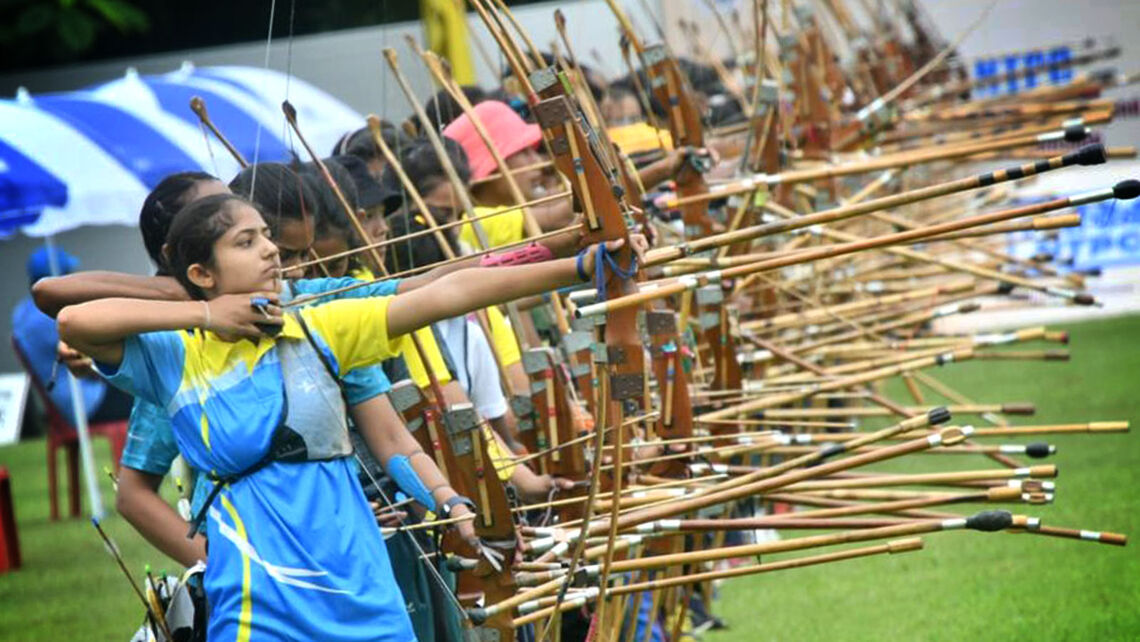This professionally taken horizontal photograph captures an archery competition featuring a diverse group of young archers, predominantly of Indian or Asian descent, standing on a lush green field. In the foreground, a girl is prominently visible, identifiable by her distinctive blue polo shirt with yellow trim and details such as a yellow collar and sleeve. She, along with her peers, is equipped with bows, arrows, finger tabs, and quivers, showcasing their readiness for the event. Numerous other children, some wearing various hats—like a black hat and a bright pink one—stand in rows behind her, aiming their blunt-tipped arrows. The depth of the row and the number of participants are difficult to ascertain due to the blurred motion of arrows in flight. Toward the side and slightly behind the archers, several white and blue tents are set up, with parents or spectators seated, including one person in a blue outfit sitting in a chair. The scene vividly captures the intensity and organization of the archery competition, highlighting both the participants and the supportive atmosphere around them.